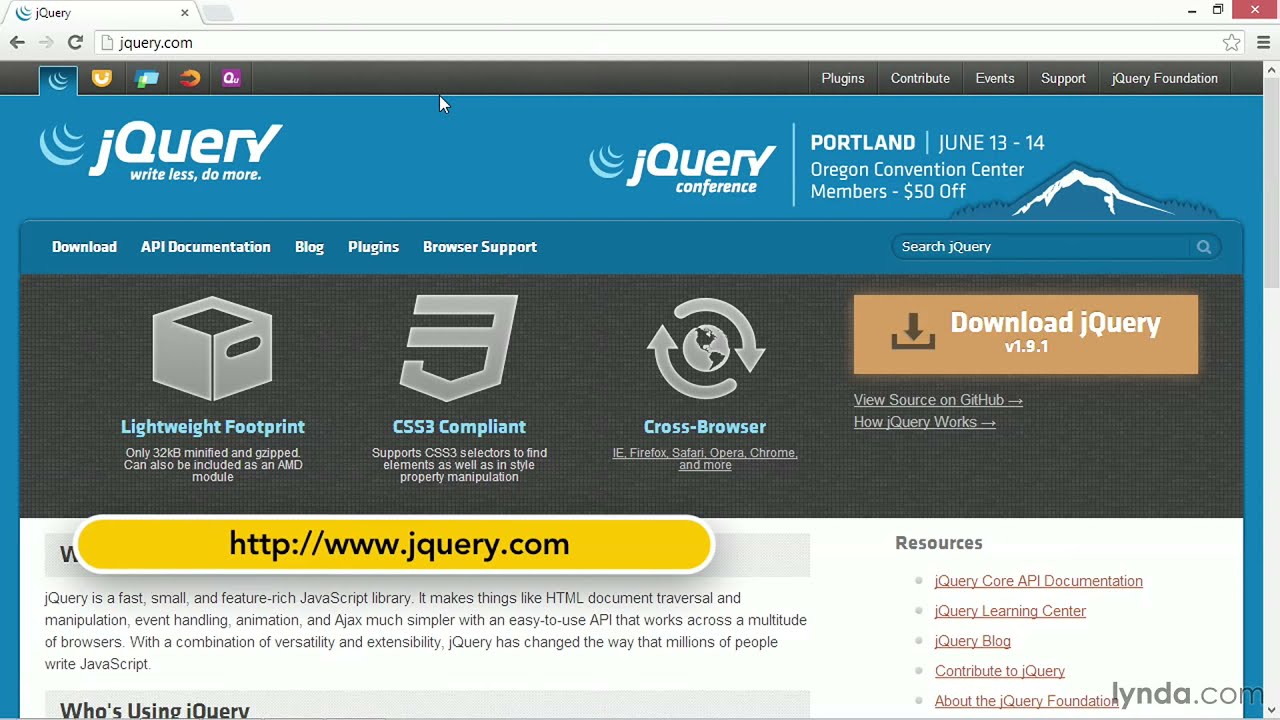A screenshot of a browser window displaying the jQuery website is shown. The browser itself has a very light gray background, and only one tab is open, labeled "jQuery" with a lowercase "j" and an uppercase "Q." The URL in the address bar is "jQuery.com."

Within the webpage, there is a narrow black border at the top, and the menu on the right side features items written in white font: Plugins, Contribute, Events, Support, and jQuery Foundation. The main header of the webpage has a blue background with the jQuery logo in white, featuring a stylized lowercase "j" and an uppercase "Q." Beneath the logo, the tagline "Write Less, Do More" is displayed in white font. To the left of the header, three light blue crescent moon shapes are arranged in a small, medium, and large sequence, creating an aesthetically pleasing image.

In the center of the page, the logo is repeated, and beneath it, the word "Conference" is written. To its right, in white font, the text reads: "Portland June 13-14, Oregon Convention Center, members $50 off," alongside a schematic drawing of a snow-capped mountain peak.

The background in the middle section of the page is dark gray. On the right side, a very light brown rectangle contains the text "Download jQuery v1.1.1" in white. Adjacent to this text is a download icon featuring a black arrow pointing to a horizontal line with tiny vertical lines on either side. Below this is a yellow rectangle with rounded corners, outlined in white. Within this rectangle, the web address "http://www.jquery.com" is written in black font.